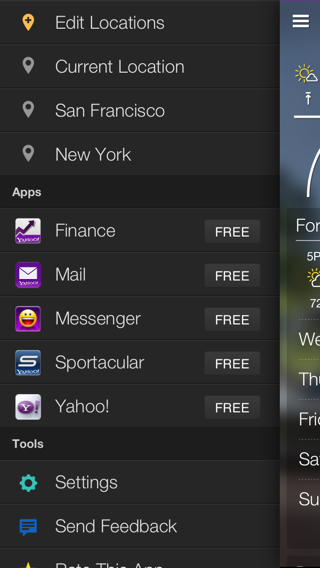The image depicts a dark-themed vertical menu interface. The background is a deep black color with sections that are a lighter shade of black, creating a subtle contrast. The topmost menu item is "Edit Locations," followed by "Current Locations." Next in the list are two location-specific entries: "San Francisco" and "New York." 

Below the location section, there is a title bar labeled "Apps," under which a list of applications is displayed. The apps listed are "Finance," "Mail," "Pass," "Messenger," "Sportacular," and "Yahoo." 

On the right side of this menu, there appears to be a partial view of a smartphone screen, showing a weather widget that provides current weather information.

The overall layout is clear and organized, with each section and item distinctly separated, making it easy for users to navigate through their options.